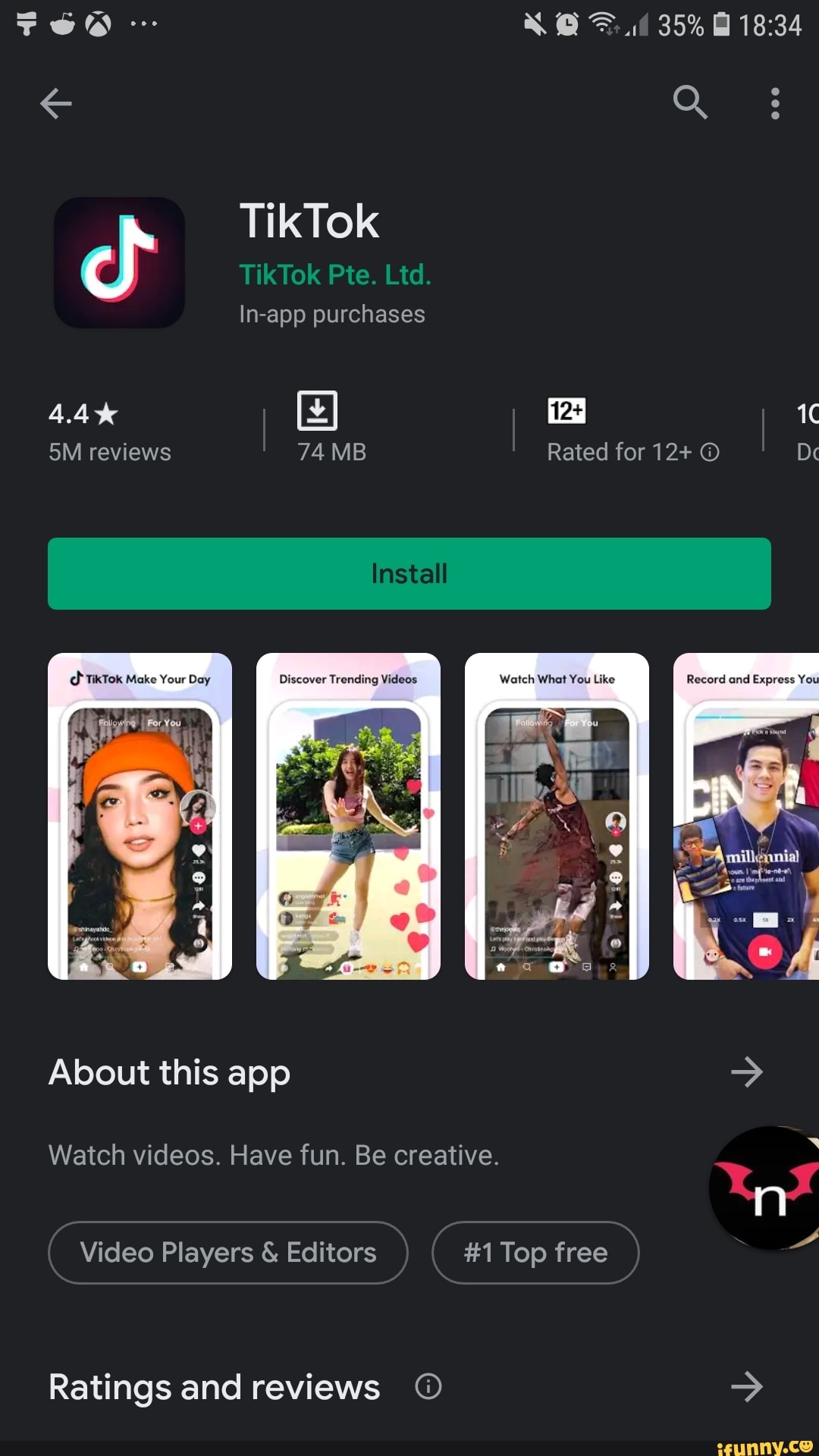The image showcases the download screen for the TikTok app on a smartphone. Prominently displayed in the center is the TikTok icon, accompanied by the app name and the producing company. The app boasts an impressive 5 million reviews and holds an average rating of 4.4 stars. The download size for TikTok is specified as 74 megabytes and the app is rated suitable for users aged 12 and above.

Positioned directly above the app details, on the right-hand side of the screen, is a small search icon. Further above, at the very top of the phone’s interface, a series of icons indicate various phone statuses: a speaker symbol, an alarm clock, Wi-Fi signal strength, cellular signal strength, and a battery indicator showing a 35% charge. The current time is displayed as 18:34.

Beneath the TikTok app details, a large, horizontal green 'Install' button invites users to download the app. Below this are four small images displaying people engaged in typical TikTok activities: a close-up of a girl’s face, a girl outdoors possibly dancing, someone scoring a basketball hoop, and a man standing outside with his hands on his hips.

Further down, there's additional information about the TikTok app and links to related video players and editing tools. This orderly arrangement provides a comprehensive overview of the app and its user community, enticing potential users with its visual appeal and accessible download instructions.